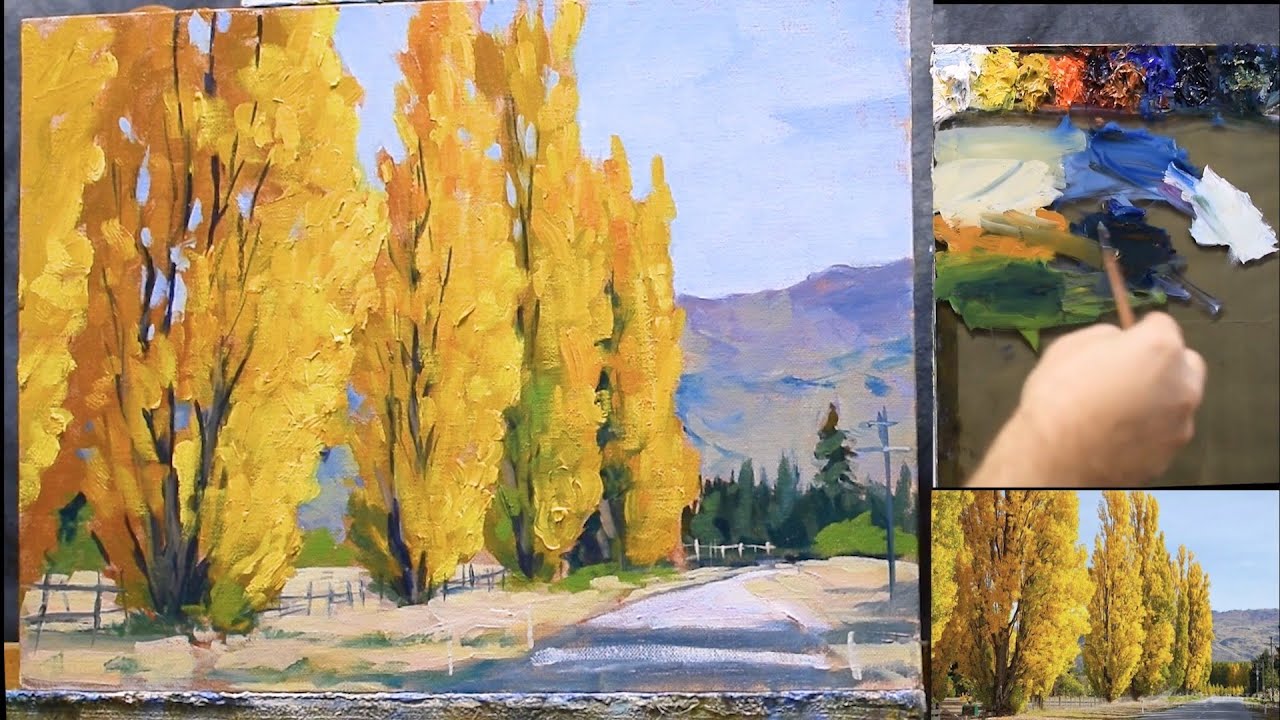The image depicts a detailed and layered artistic process. Dominating the left side is a large, vibrant painting that occupies about 75% of the space. The painting showcases a serene autumn countryside with tall, slender trees boasting golden foliage set against a backdrop of blue and purple mountains. Below the mountains are lush green forests, and a blue sky stretches over the scene. A white picket fence runs through the left side of the painting, leading to fields dotted with towering, yellow-leaved trees. To the right of the fence, a tan-brown road meanders through the landscape, with telephone poles lining its side.

On the top right, occupying around 20% of the image, a hand is seen mixing paint on a palette, seemingly in the act of creating the larger painting. Below this hand, taking up the remaining 10%, is a smaller photo that serves as the inspiration for the main painting. This photo reflects the same idyllic rural scene, complete with the yellow trees, mountainous background, and expansive blue sky, capturing the essence that the artist is meticulously recreating on canvas.